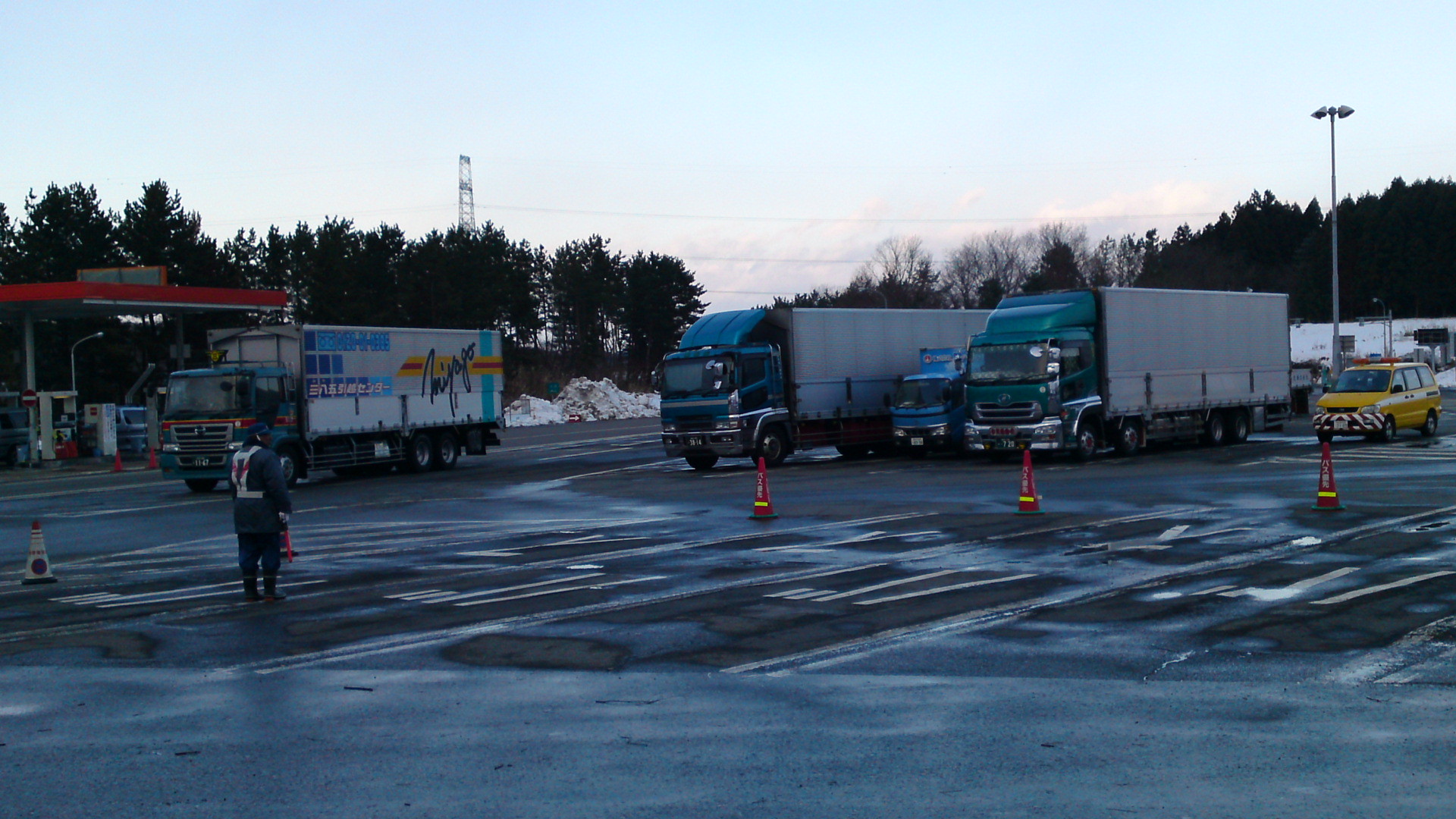The photograph captures a winter scene at a truck stop or possibly a driver training area next to a gas station. The parking lot is wet, and snow is piled up against a backdrop of evergreen trees, indicating it has recently rained or snowed. The gas station, located to the left, features a distinctive red-edged roof. In the lot, three large trucks with grey trailers and colorful cabins (one blue and one green) are parked side by side, along with a smaller light blue truck. A yellow taxi and a few other smaller vehicles are also present. A man dressed in a safety vest, heavy jacket, hat, and boots stands behind some orange cones, facing the trucks, suggesting he might be directing traffic or overseeing training. The cones line the road, possibly set up for a driver's education course. A lone truck is seen moving past the gas station, heading toward the area where the man is standing. Power lines stretch across the clear winter sky, adding to the detailed backdrop of this chilly, wet day at the truck stop.